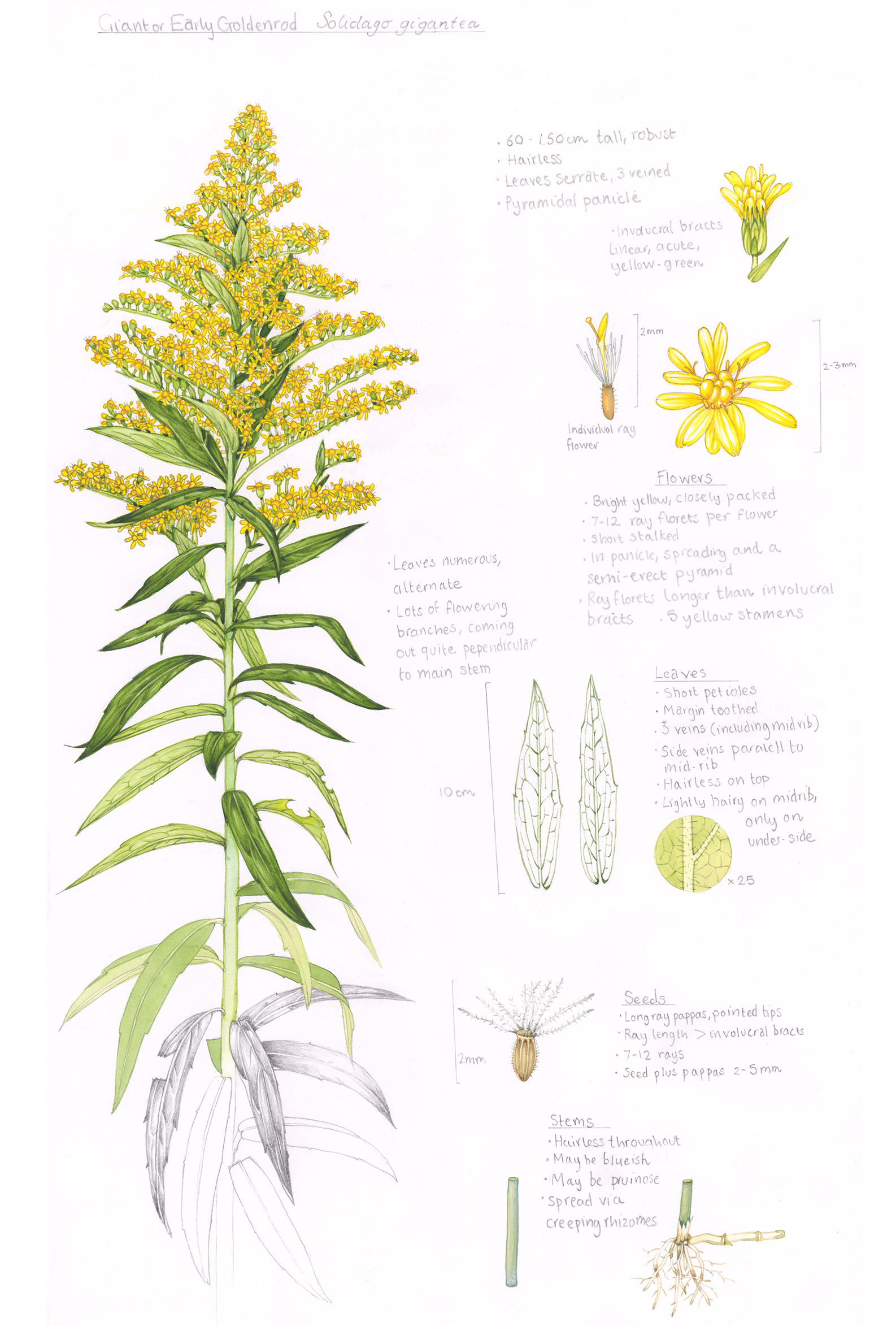The image is a detailed botanical diagram labeled "Giant or Early Goldenrod" with its Latin name, likely "Solidago gigantea," near the top. On the left side, a meticulously drawn plant showcases a progression of color from bottom to top. The base of the plant features pencil-drawn black and white leaves. As the stalk extends upwards, the leaves transition from light green to darker green. Near the top, the plant culminates in vibrant yellow flowers that densely cover the leaves, forming a point reminiscent of a Christmas tree's shape, though rounded at the peak.

On the right side, the diagram contains several components. At the top, there's a mixture of cursive and regular handwriting providing a scientific description. Beneath this, there are detailed illustrations paired with descriptions: an image of the entire flower with a green backdrop, followed by an isolated depiction of just the petals. Further down, two images outline the leaves, with a close-up circled detail of the leaf's internal structure adjacent. Additional annotations and drawings specify various parts of the plant, including the stem, flowers, leaves, seeds, and roots, with a focus on scientific measurements and characteristics. Bullet points underline key aspects of the plant, providing a comprehensive overview of the species.